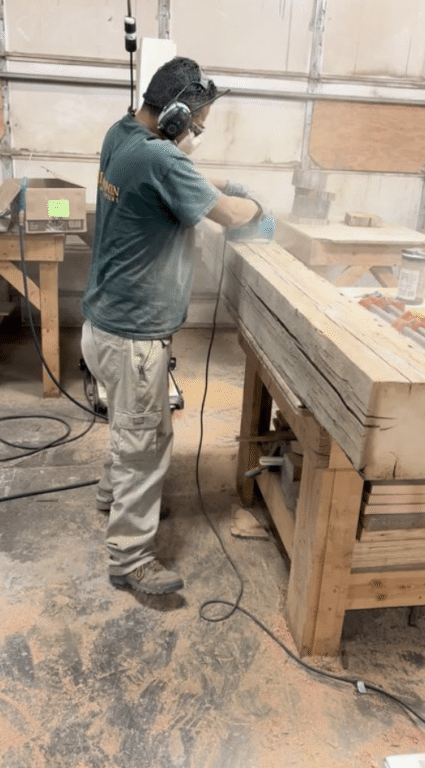The image is a vertically-oriented color photograph capturing a man engaged in woodworking. Positioned with his right side facing the viewer, he is diligently sanding a large, square piece of wood placed on a wooden workbench. The man wields a blue sanding tool, attached to which is a black cord that curls on the floor and runs off towards the bottom left side of the frame. 

In the background, there is a white wall with gray sections, resembling the back of a garage door. To the man's left and behind him, there is another wooden bench with a cardboard box on it. The man is wearing an aqua green shirt featuring yellow lettering on the back, beige khaki cargo pants, and brown work boots. He's protected with a mask and noise-canceling headphones while working. His right arm extends forward to guide the sander, and his left arm grips it from behind. 

Sawdust is visibly covering the front of his shirt and the floor is blanketed in brownish-red sawdust, indicating the intensity and focus of his labor. Something indistinct protrudes from the pocket alongside his right leg, adding to the scene's authenticity and detail.